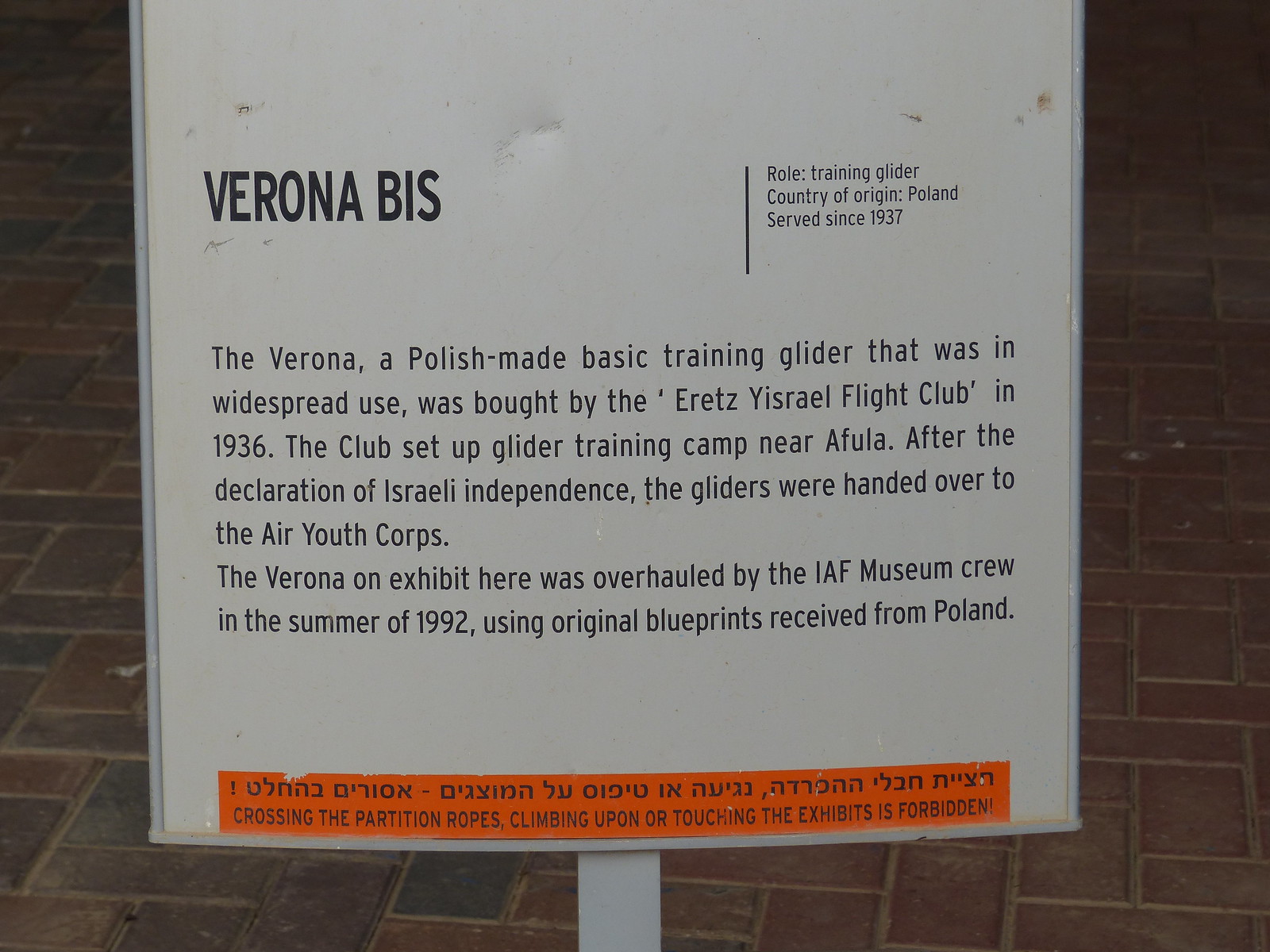In the image, we observe a white sign with a silver border positioned centrally against a backdrop of a red brick surface, which might be a sidewalk; it displays an array of reddish, purple, and darker black bricks on the left and right. The setting appears to be outdoors under daylight.

The sign bears bold black capital letters that read "Verona BIS," followed by a vertical line, and text that says “Roll Training Glider, Country of Origin Poland, served since 1937.” Below this, more details about the glider are provided:

"The Verona, a Polish-made basic training glider that was in widespread use, was bought by the Eretz Yisrael Flight Club in 1936. The club set up a glider training camp near Afula. After the declaration of Israeli independence, the gliders were handed over to the Air Youth Corps. The Verona on exhibit here was overhauled by the IAF museum crew in the summer of 1992 using original blueprints received from Poland."

At the bottom of the sign, there is an orange rectangular strip featuring some Hebrew writing. Additionally, there is a warning that reads: "Crossing the partition ropes, climbing upon, or touching the exhibits is forbidden." The colors visible in the image include white, black, orange, red, and gray.